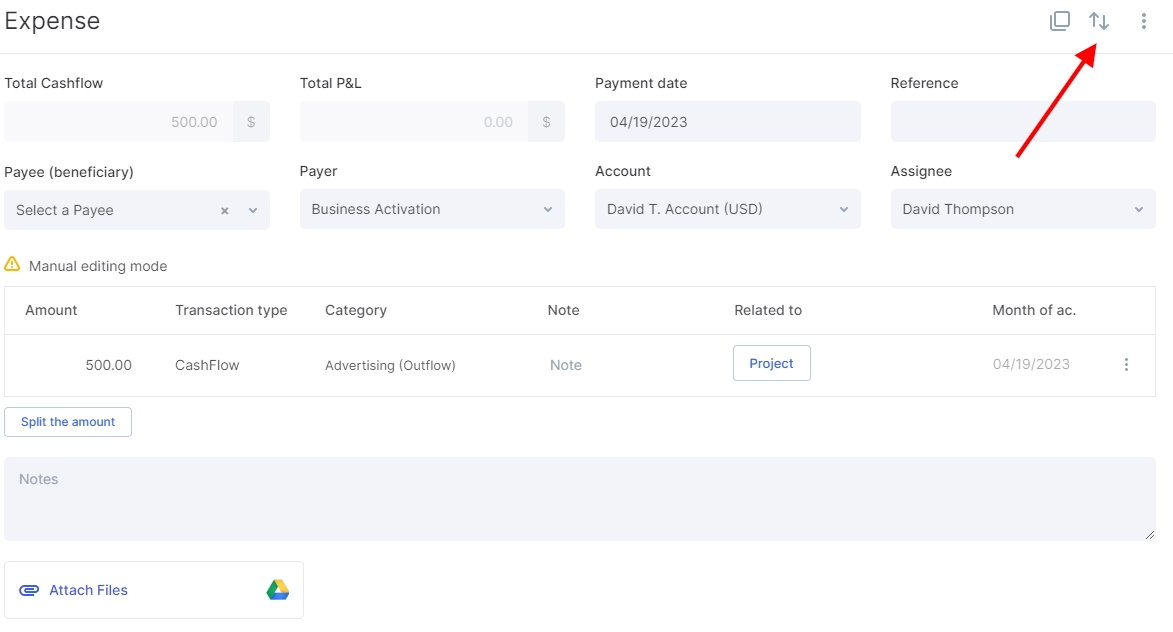The image features a white background with the word "Expense" in bold black print, starting with a capital "E" in the top left corner. To the right, there is a square icon with a shadow underneath. This icon includes up and down arrows and three vertically aligned dots. Extending downwards from the square is a thin line that connects to four distinct sections.

The sections are as follows:

1. **Total Cash Flow:** Indicated as $500.
2. **Total P&L:** Displayed as $0. "P&L" is written with a capital "P" and "L."
3. **Payment Date:** Listed as 04/19/2023.
4. **Reference:** Labeled without a specific value.

Under these sections, additional details are provided in another segmented form:

- **Payee:** Described as "Beneficiary" in parentheses, with a prompt to "Select Payee."
- **Payer:** Labeled as "Business Activation."
- **Account:** Named "David T account" and specified to be in "US dollars."
- **Assignee:** Mentioned as "David Thompson."
- **Mode:** Indicated to be in "Manual Editing."
- **Amount:** The transaction amount is not specified here.
- **Transaction Type:** Not mentioned in the given text.
- **Category:** Not explicitly mentioned.
- **Note:** Related to the month of AC (implied, but not expanded upon).
- **Amount Split:** Implied to be an option, but specifics are not given.
- **Additional Notes:** Not detailed in the given text.
- **Attached Files:** Noted as an option but not specified further.

The image appears to be a detailed expense management interface, showing various financial details and organizational fields relevant to documenting and processing expenses.